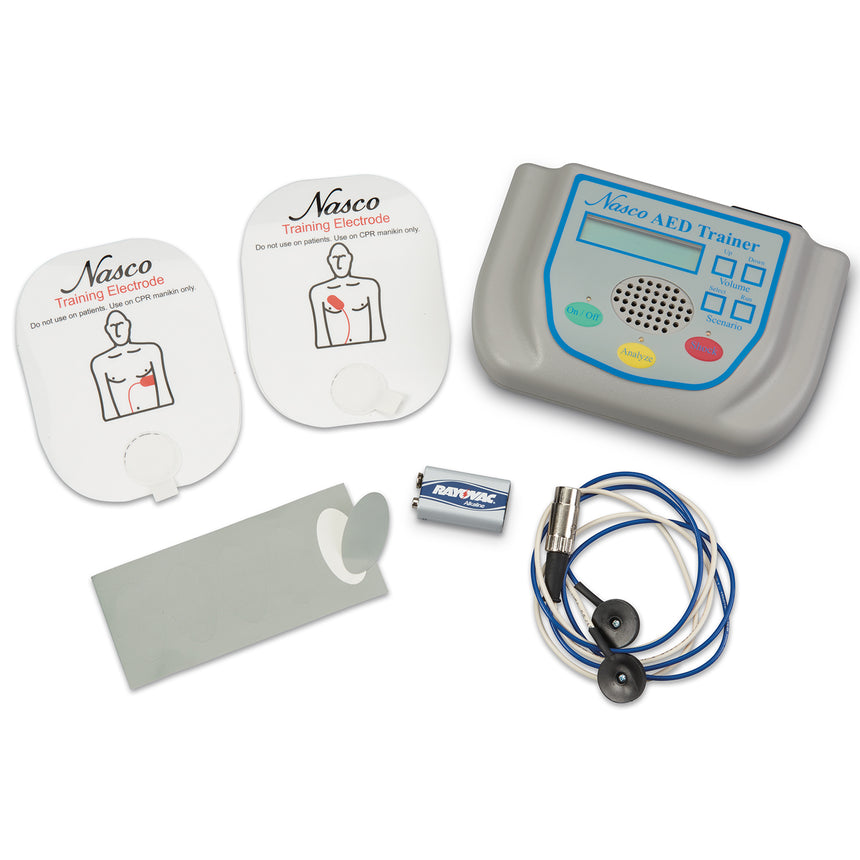The image showcases various components of a NASCO AED trainer, specifically designed for educational and training purposes. Dominating the top row are two white training electrode pads, each displaying an illustration of a bald man from the waist up with a red pad placed on his left and right chest areas respectively. Both pads are labeled "NASCO Training Electrode" in prominent black and red lettering. Adjacent to the pads on the right, there is a gray control box labeled "NASCO AED Trainer" in blue lettering. This device features a small screen, a central speaker, and various control buttons with green, yellow, and red indicators. Below this control box, there is a flat, gray panel. The bottom row contains a gray Rayovac battery with blue trim, lying sideways, and a set of electrodes with blue and white wires, ending in black-tipped connectors. These components, including the electrode wires and suction cup-like stoppers, are integral to the AED training process, simulating the attachment and functionality of a real medical device used for cardiac emergencies.